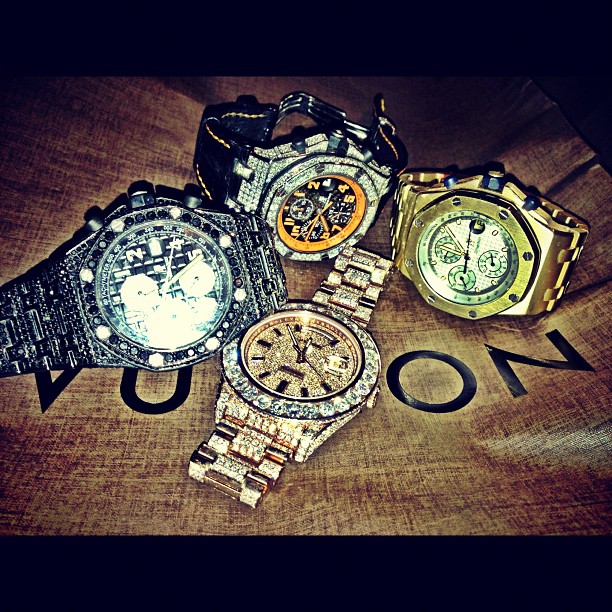This photograph showcases a collection of four opulent, jeweled watches arranged on a surface that seems to be a flexible Louis Vuitton tote bag. The surface features partially visible letters "B-U-I-T-T-O-N," indicating it spells out "Vuitton." The bag is a brown color with black lettering. The overall composition is quite detailed, drawing attention to the luxurious and expensive nature of the timepieces.

Starting from the bottom left and moving clockwise, the first watch is predominantly gold with a thinner band, suggesting a style more fitting for women. Its bezel and watch face are encrusted with diamonds or diamond-like crystals. Moving on, the second watch has a darker appearance with black stones around the bezel, although its face is somewhat obscured by a reflection. At the top, a more contemporary piece stands out with its black nylon band adorned with orange accents, black bezel, and encrusted gems, featuring orange numerals on a black dial. Lastly, the fourth watch on the right, chunkier in design, is also gold but lacks any gems.

In summary, this indoor photo captures four distinct, ornate watches, each lavishly appointed with precious stones and varying metallic finishes, resting elegantly on what is unmistakably a Louis Vuitton surface.